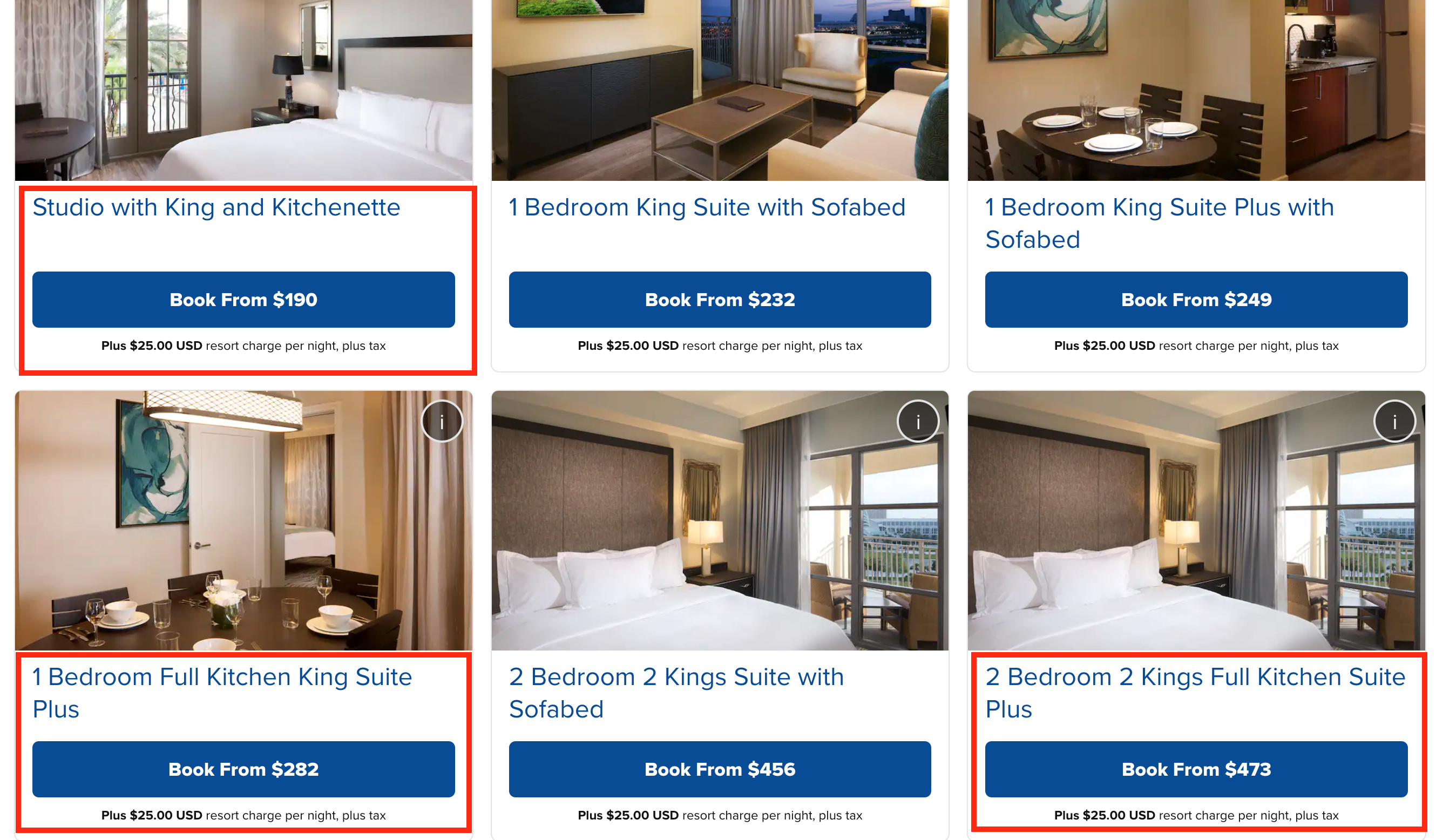This image depicts a room booking webpage showcasing various studio apartments and hotel room options. Three specific accommodations are highlighted with red rectangles:

1. In the upper left corner, a "Studio with King and Kitchenette" is offered from $190 per night, accompanied by a $25 USD resort charge plus tax. The room features a bed adorned with crisp white linens, a lamp, and a view from a balcony.

2. Directly below it, a "One Bedroom, Full Kitchen, King Suite Plus" is available, starting at $282 per night. 

3. In the lower right corner, a "Two Bedroom, Two Kings, Full Kitchen Suite Plus" is highlighted, starting at $473 per night, plus the same $25 USD resort charge and taxes. 

Additionally, a similar suite to the two-bedroom option is listed in the middle, priced slightly lower at $456 per night. The webpage appears to be a platform for booking these various types of accommodations, possibly servicing studio apartments, hotel rooms, or Airbnbs.